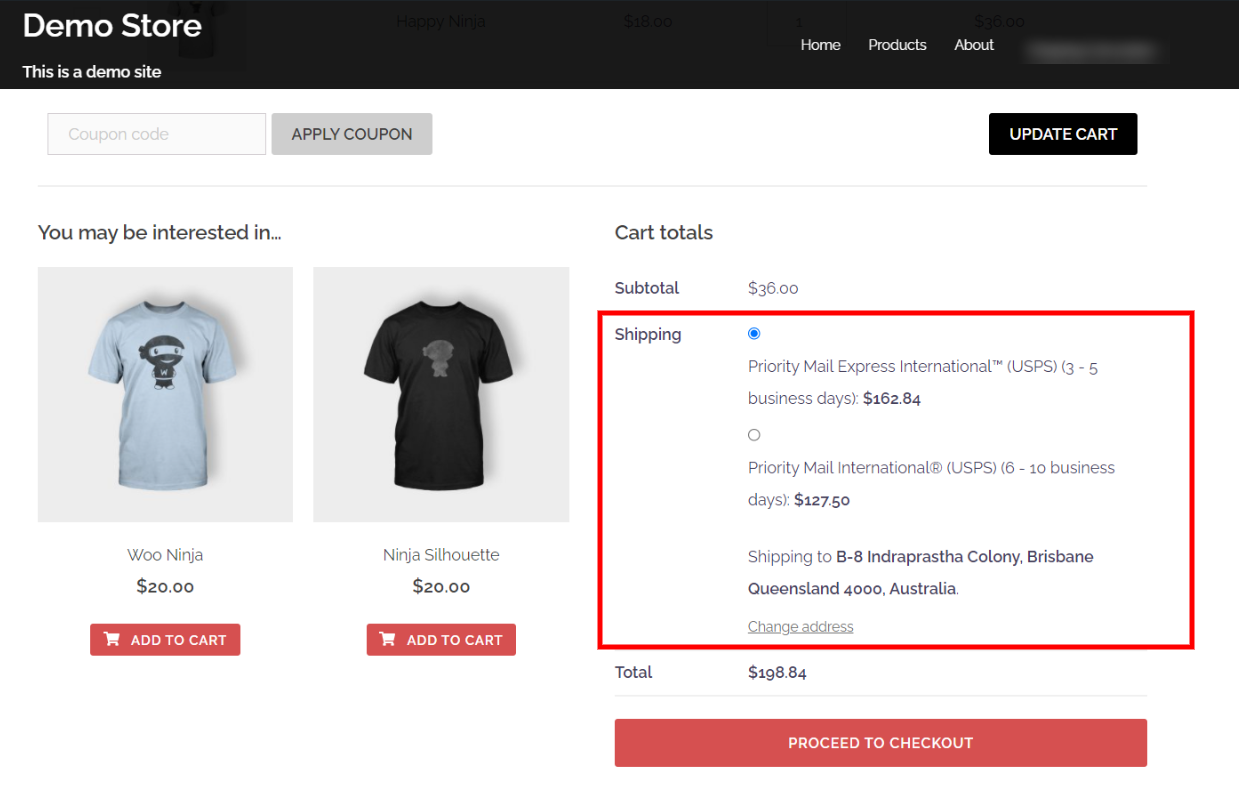The image depicts an online store interface labeled "Demo Store" in the upper left corner, with the text "This is a demo site" positioned beneath it. On the top-right corner, there is a navigation menu that includes options for Home, Products, and About, although some part of it is obscured.

Below the black navigation bar, which features white text, there is a section for applying a coupon code. This section includes a gray input box outlined in gray for entering the code, accompanied by a gray button with black text that reads "Apply Coupon." Adjacent to this area is another button labeled "Update Cart," which is black with white text.

The main content showcases two T-shirts available for purchase. The first is a gray T-shirt featuring a cartoon ninja, priced at $20, under a title "Woo Ninja." Below this item is a red "Add to Cart" button with a white cart icon and text. The second item is a black T-shirt with a ninja silhouette, also priced at $20, with a similar "Add to Cart" button.

At the bottom, the "Cart Totals" section provides a summary, showing a subtotal of $30. It includes detailed shipping options, with "Priority Mail, Express International, USPS, 3 to 5 business days" selected. This option is indicated by a blue-filled selection circle and is outlined in red, with a shipping cost of $162.84.

The overall layout is clean and user-friendly, providing clear options for navigation, product details, cart management, and shipping information.